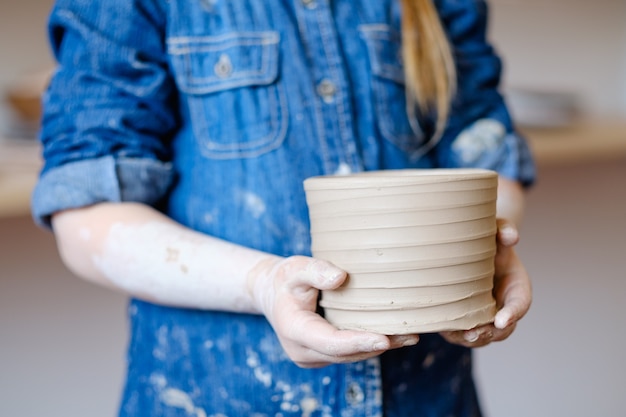This indoor photograph captures a woman displaying her pottery creation. She is centered in the frame, facing slightly to her right, with the image showing her from the mid-hip to just below the shoulders. The overall photo is slightly blurry, with sharp detail on her hands and the pottery she holds. She is dressed in a messy, long-sleeved blue jean shirt with rolled-up sleeves, revealing some splattered stains likely from her pottery work. The shirt features pockets on both sides of the chest. Her blonde hair, tied in a ponytail, cascades over her left shoulder. She holds a light tan, handcrafted clay pot with both hands, suggesting recent participation in a pottery class. The background is blurred, showing a gray floor and a lighter upper wall with some brown elements, possibly a bench area. The image measures approximately five inches wide and three inches high, framing a close-up view of her pottery creation.